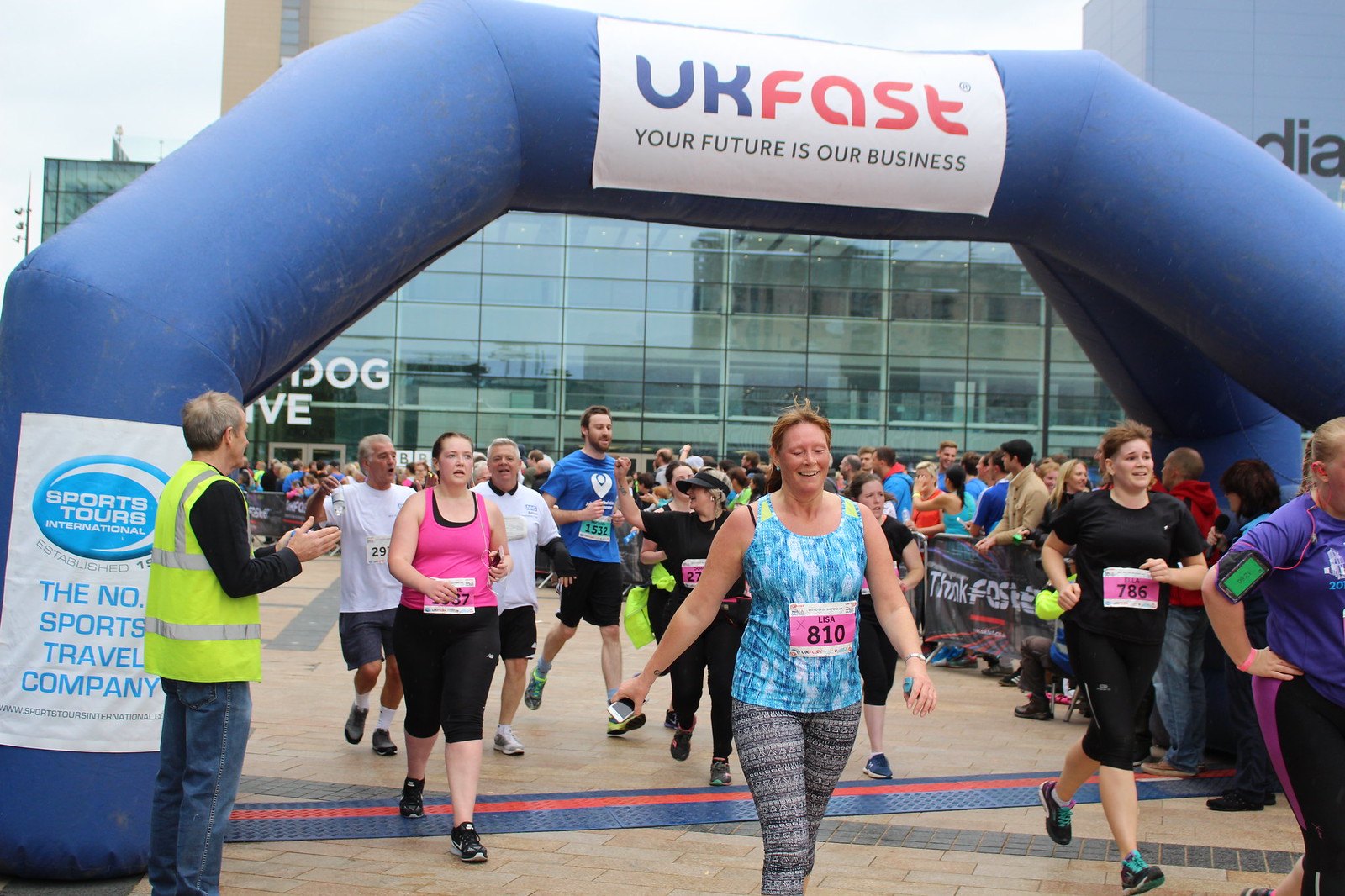This photograph captures a lively outdoor charity event, possibly a 5K walk or marathon, featuring numerous participants adorned in workout apparel with pink and white bibs bearing their numbers. The focal point is a striking blue inflatable archway inscribed with "UK FAST, your future is our business," accentuated with "UK" in blue and "FAST" in orange. Beneath the arch, participants, who range in age and gender, are energetically walking or running across a red finish line drawn on the ground. To the side, a race worker in a black long-sleeve shirt and neon yellow safety vest is enthusiastically clapping for the participants. Surrounding the scene are spectators cheering them on, adding to the celebratory atmosphere. In the background, a large glass building towers over the event, with snippets of blue sky visible, framing this moment of community and achievement.